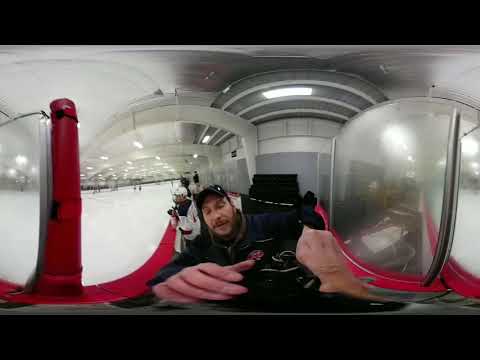In this extreme wide-angle panoramic shot, we are positioned in a booth outside an indoor ice rink. Dominating the foreground is a middle-aged man, possibly in his 40s, wearing a black baseball cap, dark blue jacket, and goggles, with a mustache and closed eyes. He is taking a selfie, with his right hand visibly holding a camera or another device towards himself. The man is framed by curved glass windows featuring red stanchions on either side.

Behind him, a hockey game appears to be underway, though the panoramic distortion makes the players and their actions seem distant and tiny. A hockey player in a white and blue uniform with a white helmet stands at the red railing, observing the ice. The rink is brightly lit, with lights on the ceiling and in the audience area. The ice itself is dotted with several skaters, adding a sense of depth to the background scene. The overall image effectively captures the bustling, albeit slightly distorted, activity at the rink.